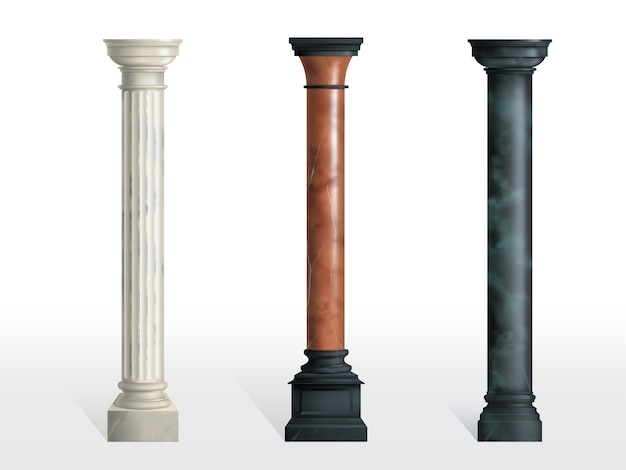This image is a highly detailed, textbook-like photograph showcasing three distinct styles of architectural columns, set against a crisp white background with a corresponding white floor. The first column on the left is reminiscent of the classic Roman Colosseum style, featuring a predominantly white, vertically beveled surface with subtle gray variegations, suggesting it is crafted from stone or marble. The central column stands out with a unique appearance combining materials and colors: the shaft is an orange-bronze or copper hue with delicate gradients, flanked by a black iron top and base, possibly hinting at influences of both metal and wood construction. Lastly, the third column on the right exhibits a dark gray, almost black, stony texture, with a gradient overlay suggestive of dark blue shades, terminating in square bases and tops, but maintaining a rounded shaft. Each column casts distinct shadows, enhancing the image's depth, impressionistic of a computer or AI-generated illustration often found in educational materials.